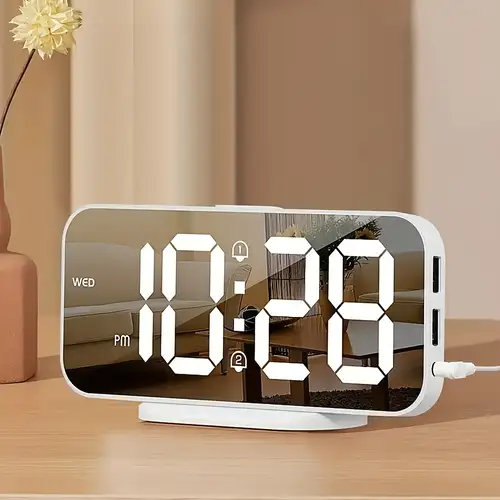This meticulously crafted artwork presents a hyper-realistic scene centered around a horizontally positioned white smartphone, serving as a creative clock. The phone, ensconced in a matching white stand, rests atop a wooden table. Displayed prominently on its screen in large white digital text are the time "10:28 PM" and the day "WED." Flanking the digits "10" and "28" are icons indicating two alarms. The screen also reflects the surrounding room, revealing a cozy living space with a coffee table, couch, plant, and a balcony in the background. Connected to the phone is a white cable, suggesting it's being charged. To the left of the phone, a flower with a yellow bloom emerges from a clay vase, adding a touch of nature to the scene. This setup is framed against a backdrop of beige and brown walls, lending a warm and inviting ambiance to the overall composition.